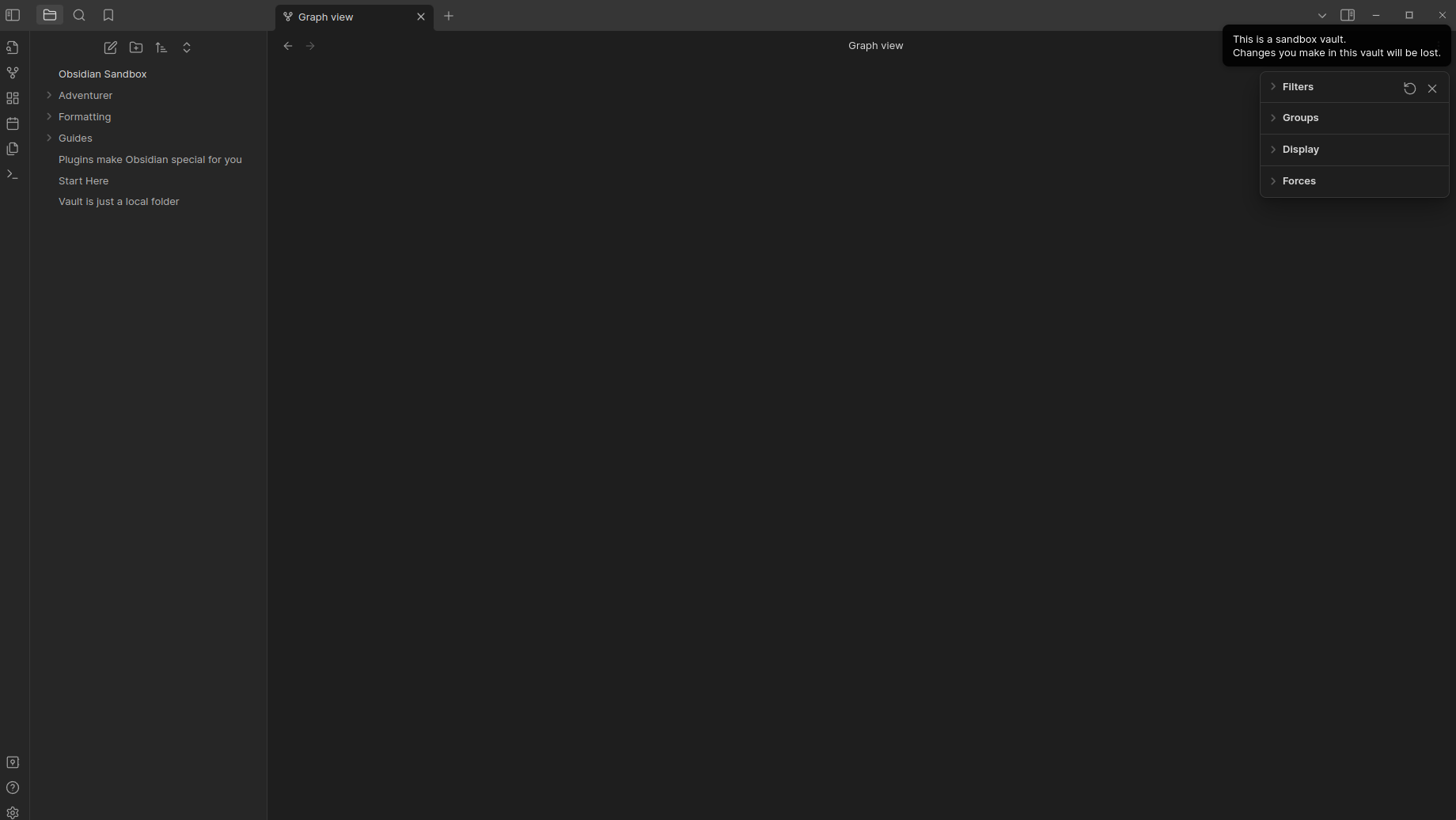The image depicts an interface with a dark gray background, potentially representing an API or similar software tool. On the left side, there is a prominent sidebar titled "Obsidian Sandbox," organized into several tabs. The top tab is labeled "Adventure," followed by another tab named "Formatting." On the right side of the interface, there are additional tabs for further customization and management, including "Filters," "Groups," "Display," and "Forecast," with the "Forecast" tab appearing at the bottom in white text.